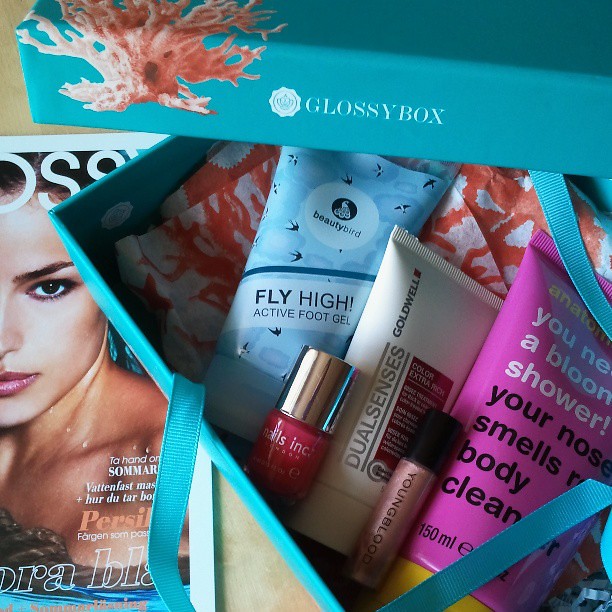The image features an assortment of beauty products placed within a blue glossy box. The box's lid, positioned at the top right corner, is teal with white text stating "Glossy Box" and a design of peach-colored coral. Embedded within the box is a collection of various products cushioned by white and orange crepe paper. A light blue tube labeled "Fly High Active Foot Gel" from Beauty Bird Company can be seen prominently along with a bright pink nail polish by Nails Inc., which has a gold top. Adjacent to this is a darker lip gloss with a black cap. There’s also a white tube labeled "Goldwell Dualsenses Color Extra Rich." Additionally, a bright pink tube marked "Anatomy You Need a Bloom Shower Your Nose Smells Body Clean" stands out. On the table to the left of the box, partially covered by the box, lies the cover of a fashion magazine. The magazine's cover features the face of a very young woman emerging from water, showing only her shoulders and face.